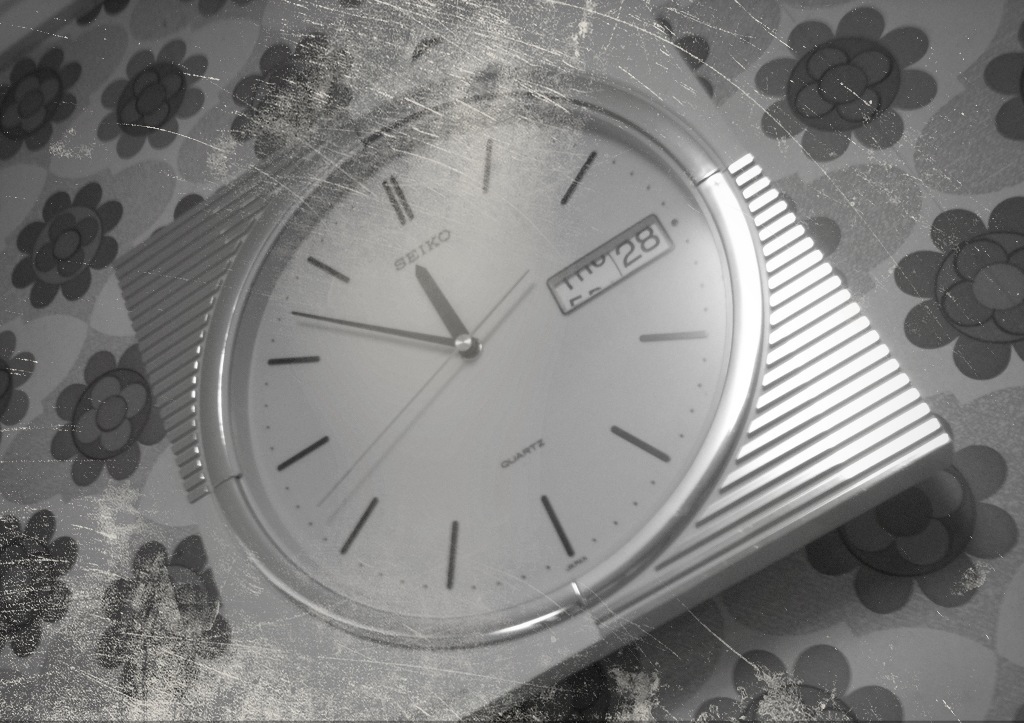This detailed caption depicts a close-up image of a silver-colored clock or watch face. The clock displays the date as Thursday, February 28th, and the time is seven minutes to noon. The face of the clock is white and features a large circular design. The clock face is adorned with raised square lines and is encased in a silver frame. The image appears slightly faded at the bottom left-hand side where there are visible scratches. The clock or watch rests on a gray and white tablecloth that is decorated with floral patterns. The flowers on the tablecloth are rendered in varying shades of gray and are detailed with black circles, but lack any additional color.